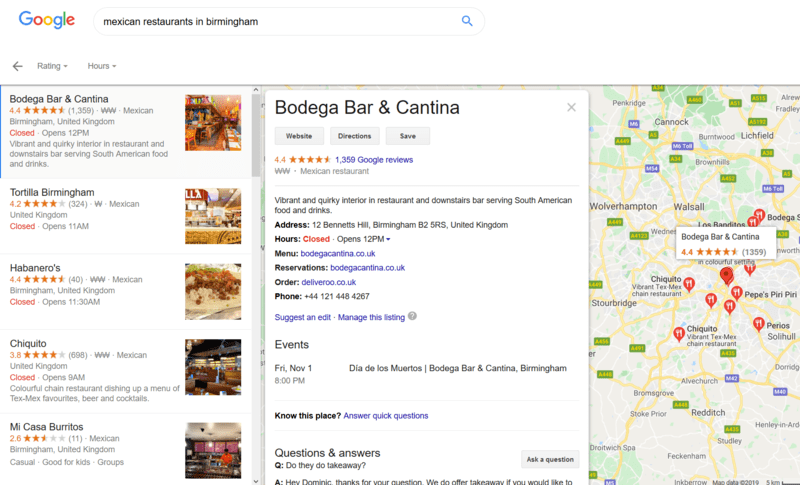This image shows a Google search result page for "Mexican restaurants in Birmingham," with detailed listings on the left side of the screen. The typed query appears in black inside the search box at the top.

The search results display five Mexican restaurants, with information on ratings, opening hours, and additional details:

1. **Bodega Bar and Cantina**: Highly rated with 4.4 stars. Currently closed and will open at 12 PM. It boasts the highest number of reviews, standing at 1,359. The restaurant features a vibrant and quirky interior, both in the dining area and the downstairs bar, and serves South American food and drinks. It is located at 12 Bennetts Hill, Birmingham, B2 5RS, United Kingdom. It opens at 12 PM and offers options for viewing the menu, making reservations, and ordering delivery. Contact number: 444-121-448-4267. Notably, they are hosting a "Dia de los Muertos" (Day of the Dead) event on November 1st, starting at 8 PM.

2. **Tortilla, Birmingham**: Rated 4.2 stars out of 5. Will open at 11 AM.

3. **Habaneros**: Also enjoys a 4.4-star rating and will open at 11:30 AM.

4. **Chiquito**: Carries a 3.8-star rating and opens early at 9 AM.

5. **Mi Casa Burritos**: Has a lower rating of 2.6 stars out of 5, with no opening hours provided.

The map feature on the right side of the screen shows the location of these restaurants, with Bodega Bar and Cantina currently highlighted as the top choice.